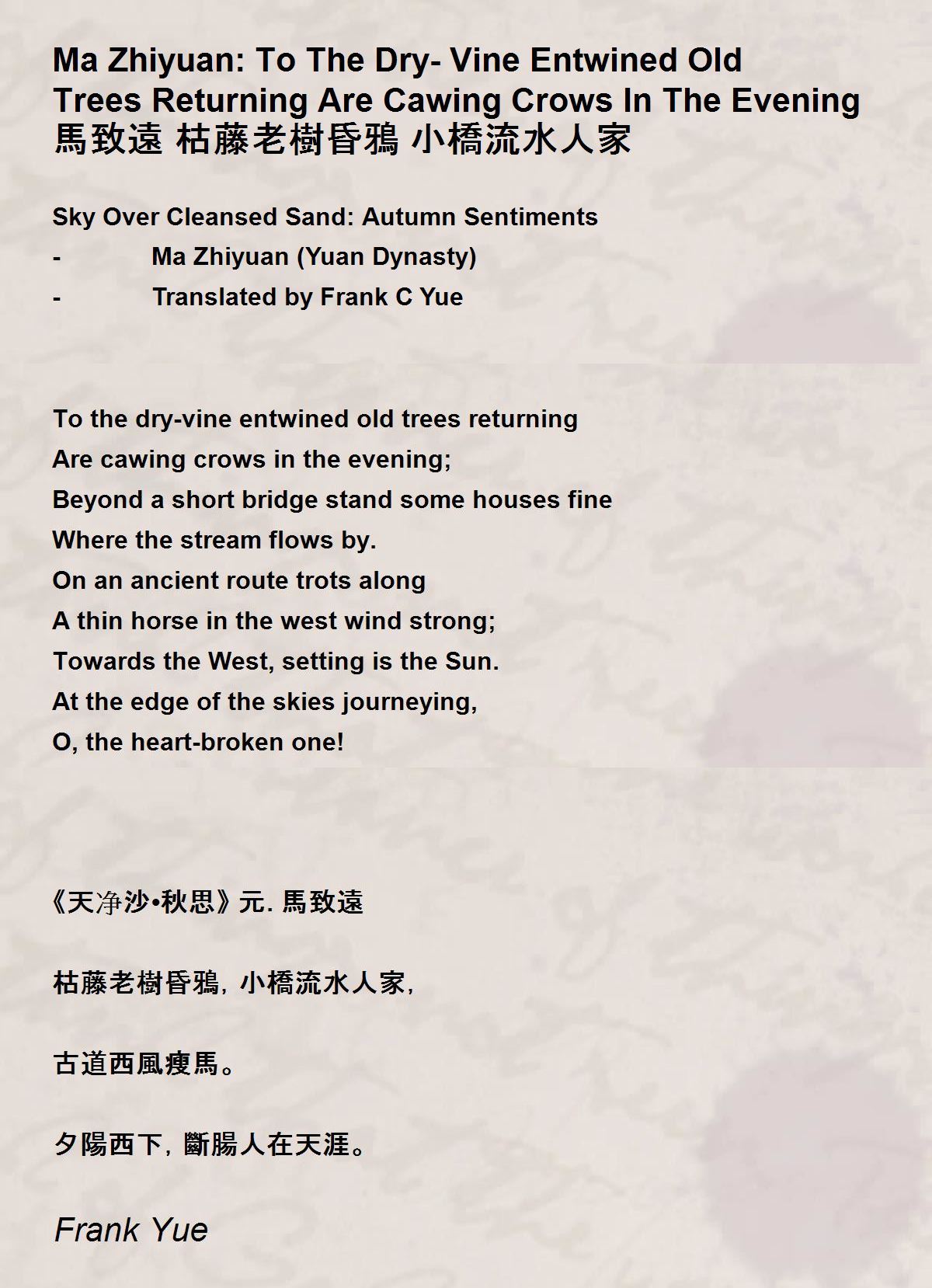The image features a densely packed text page presenting a poem in both English and Chinese, set against a white background that includes faint cursive script as a design element. At the top in bold black text, it reads "MA ZHONG," followed by the English translation of a Chinese poem: "To the dry vine entwined old trees, returning are calling crows in the evening. Beyond a short bridge, a woven stone, a house stands fine, where the stream flows by; on an ancient road, travels a thin horse in the western strong wind, towards the west setting sun at the horizon. Oh, the heartbroken one." The translation is attributed to Frank C. Yu, whose name appears at the bottom in thinner black lettering. The poem itself occupies a central place on the page in big, bold black lettering, with accompanying Chinese text positioned both above and below the English translation. This multifaceted presentation adds an interesting layer to the image, showcasing the depth and cultural blend of this literary piece.